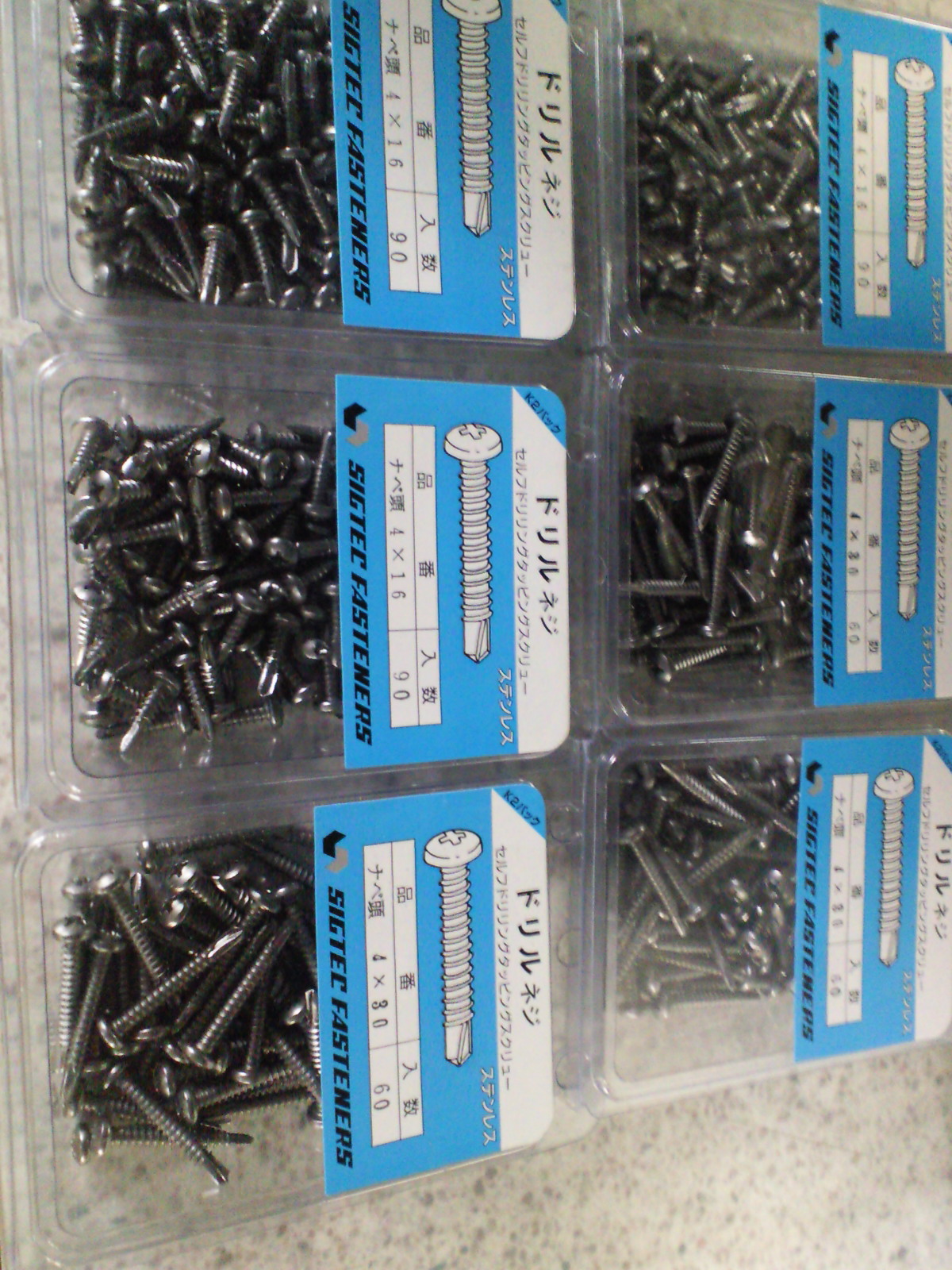The image captures six white plastic containers of screws, each neatly arranged in two rows on a gray and white marble surface. The transparent boxes reveal shiny, silver screws inside, with an estimated 50 screws per container. The screws vary in size, featuring common dimensions such as 4x16 and 4x30, typically used for applications like drywall pinning. The packaging is uniformly labeled with blue and white tags, featuring black font, and prominently displays the brand name "Sig Tech Fasteners" in English, although much of the writing is in an Asian script that cannot be read. The packages appear unopened, and the screws have a new and pristine appearance. The perspective of the photograph is slightly tilted to the left, offering a detailed view of the containers and their contents.